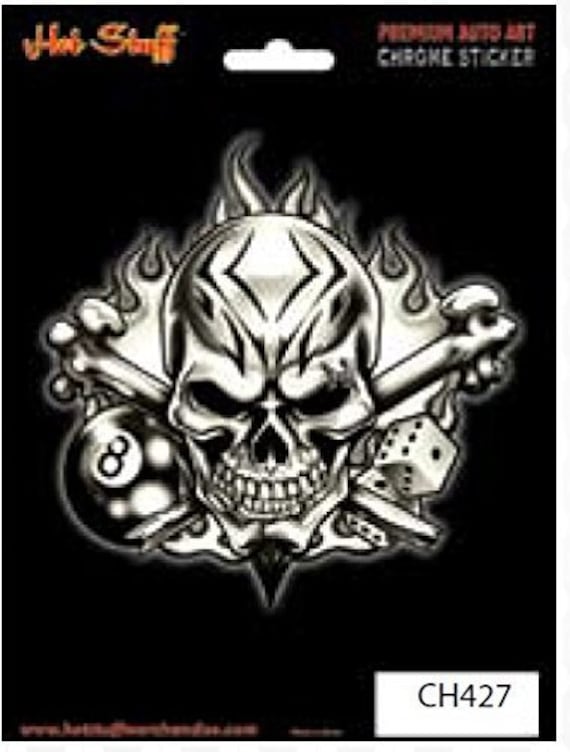This image, which likely depicts a store item, is rectangular, measuring approximately six inches high and four inches wide. Despite its overall blurriness, various details can still be discerned. The background is plain black, and at the top center is a small white keyhole cutout, designed for hanging the item on a store hook.

In the upper left-hand corner, the text "Hot Stuff" is written in a bright reddish-orange, cursive font. To the right of this is another set of text spanning two lines; the first line is in red and too blurry to decipher, while the second line, in white font, reads "CH Chrome Sticker" or simply "chrome sticker." The sticker itself occupies the center of the image and is a silver and black depiction of a skull with a knife in its teeth, crossbones behind it, flames above its head, an eight ball to the left, and a pair of dice to the right.

In the lower corners, more text is barely legible due to the blurriness. In the lower left corner, there is a streak of unreadable red print, possibly a website or contact information. The lower right corner features a white rectangular box that clearly states "CH427" in black font, one of the clearest elements in this otherwise fuzzy image.